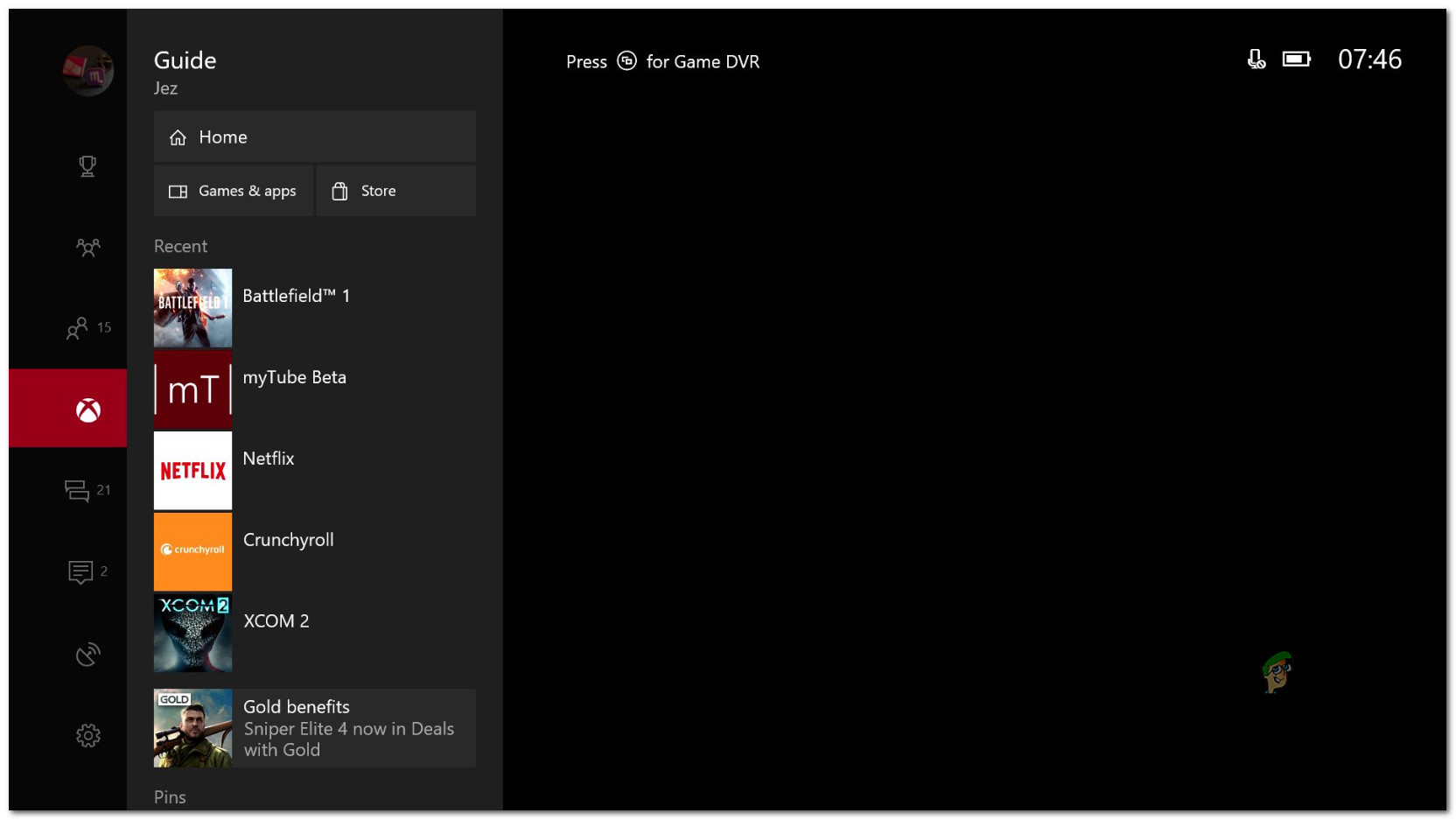The image features a predominantly black background. At the top of the screen, there's a dark gray pop-up labeled "Guide" in white text. Below this pop-up, the background lightens slightly to a charcoal shade. This section displays several menu items in white text: "Home," "Games & Apps," and "Store," which is accompanied by a shopping bag icon.

Further down the screen, various icons are visible, each with corresponding text in white. These icons include: "Battlefield 1," "My 2 Beta," "Netflix," "Crunchyroll," "XCOM 2," and "Gold Benefits." Adjacent to these names, there is an instruction to "Press," followed by an illustration of a small circle featuring two tiny squares inside it, indicating the Game DVR (Digital Video Recorder) functionality.

On the right side of the screen, a battery icon is displayed along with the current time, "07:46," both in white text. 

In the background, behind the guide pop-up, additional icons are subtly visible. At the top is a circle with intricate graphics resembling small blocks. Moving downwards, there is a trophy icon, an icon representing people labeled "15," a red square icon with an "X" inside, followed by the numbers "21," "2," and finally, a settings gear icon at the bottom.